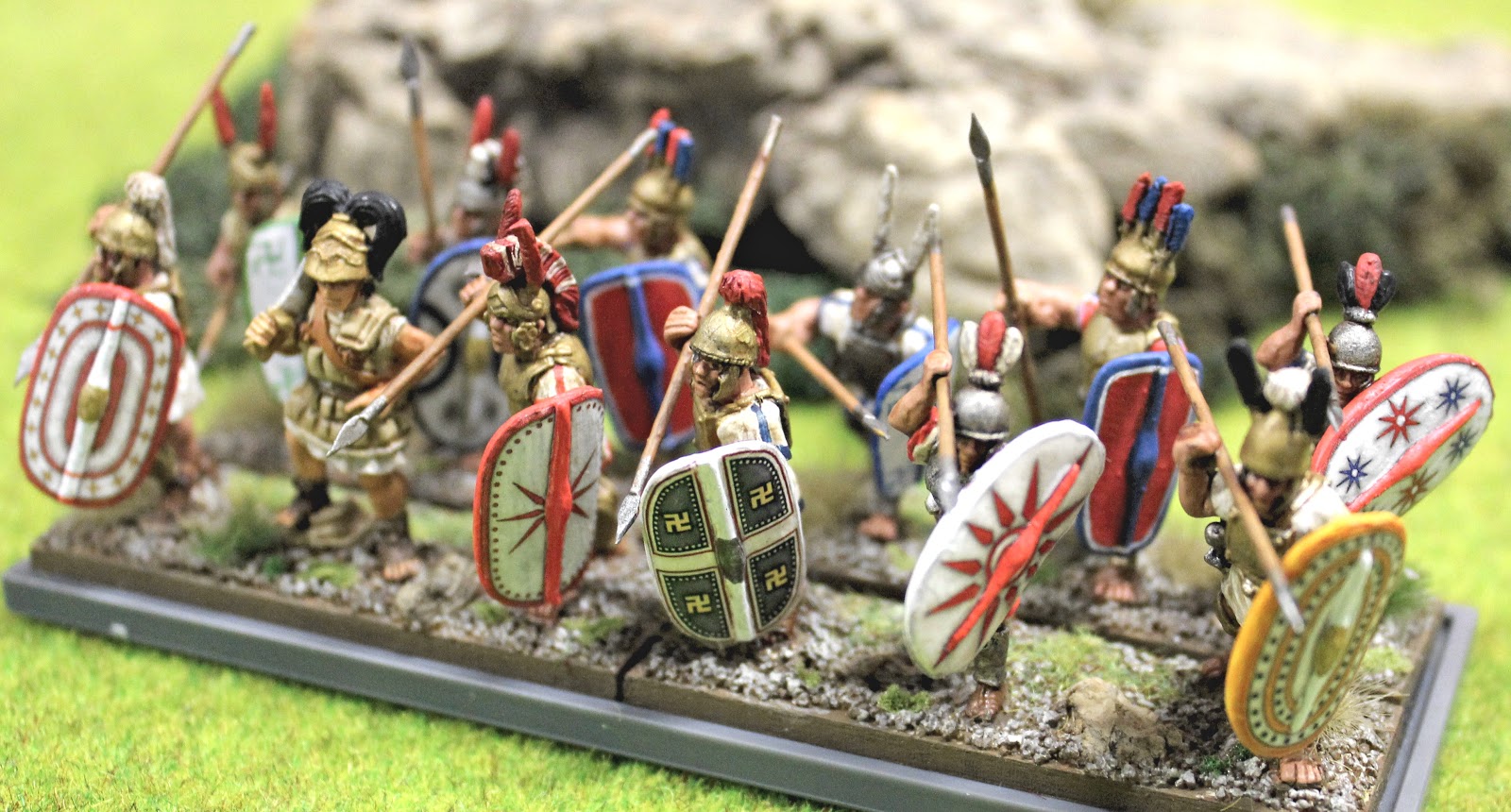This is a detailed close-up photograph of miniature toy Roman soldiers arranged on a plastic tray covered with fake grass and soil. The setting appears to be indoors. The scene showcases around seven soldiers, predominantly equipped with shields and long spears, which they hold ready for combat. Almost all the soldiers sport the distinctive red plume typical of ancient Roman helmets, adding a touch of historical authenticity.

Going from left to right, the miniatures are meticulously detailed:
1. A soldier with a red and white shield.
2. Another in armor and a helmet, holding what appears to be a hammer.
3. A soldier with a red and white shield and a helmet, brandishing a spear.
4. A man with a green and white shield and helmet, also wielding a spear.
5. A soldier with a red and white plume, a red and white shield, and a spear.
6. A soldier carrying a gold helmet, a yellow and white shield, holding a spear.

Some soldiers in the background can be seen out of focus, one with a silver armor and a spear, another with a gold armor and a red and blue plume, and a few others with spears held aloft.

The shields display various designs, including one that resembles a backward swastika, another with a sun design, and others featuring different color patterns, adding to the diversity and intricacy of the scene. The background includes toy rocks, enhancing the battle tableau.

Overall, the image captures a small yet vivid scene of ancient warfare, with a strong emphasis on the Roman legionnaires poised for action on a lifelike terrain.